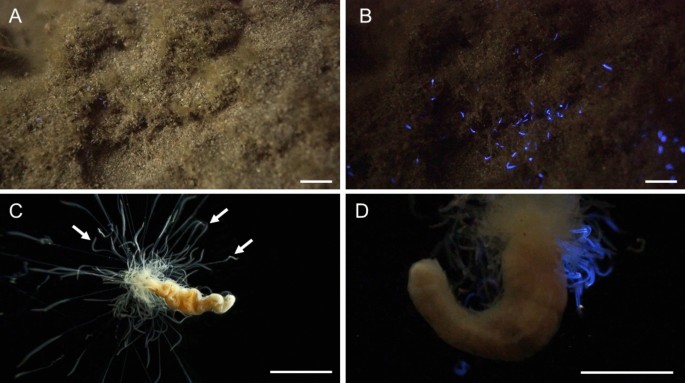The horizontally aligned rectangular composite image is divided into four sections, each labeled with an uppercase letter (A, B, C, and D) in white. The divisions are marked by white strips running horizontally and vertically through the center. 

Starting with the upper left corner, labeled A, this picture displays a well-lit brown bumpy surface, possibly resembling land or an underwater scene with clumps that could be sand or dirt. Moving to the right, picture B maintains the same brown surface but set against a very dark background. This scene is accented by tiny fluorescent blue specks, suggesting an observation of the surface under a different light, revealing glowing features.

In the lower left corner, labeled C, the image showcases a long, spiraling, tan-colored structure with numerous fibrous projections. The background here is solid black, and white arrows point towards the structure, which appears worm-like with a resemblance to spaghetti-like projections. The final image, D, in the lower right, provides a close-up view of the same worm-like structure seen in C. It’s now more curved, akin to a piece of shrimp, and features additional highlighted blue, squiggly lines with fibers, all against a black background.

Collectively, the images depict microscopic views of various structures, transitioning from a broad surface study to detailed examinations, illuminated under different lighting conditions to reveal their intricate, glowing features.